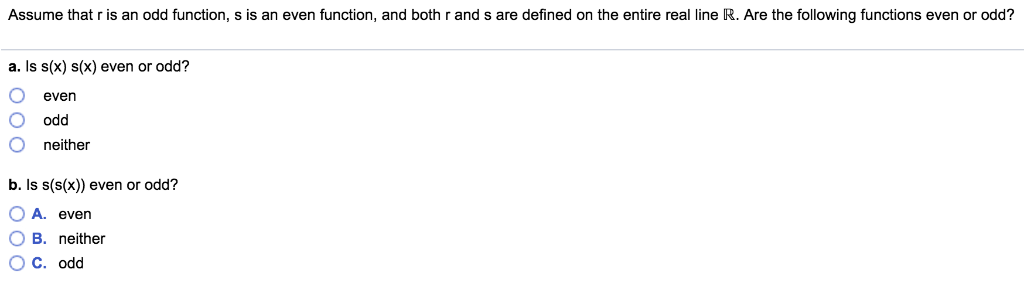This screenshot captures an image of a test question formatted in black and white. The prompt begins with a brief overview: "Assume that R is an odd function and S is an even function, both defined over the entire real line, \(\mathbb{R}\)." The question seeks to determine whether the subsequent functions are even, odd, or neither.

Part A asks: "Is \(S(x)\) even or odd?" Below this question are clickable options in the form of blue circles:
- "Even"
- "Odd"
- "Neither"

Part B poses a similar question: "Is \(S(S(x))\) even or odd?" The options for this part appear as blue circles labeled with capital letters followed by periods:
- A. "Even"
- B. "Neither"
- C. "Odd"

Each circle is clickable, designed to be filled in when selected. This structure suggests an interactive test format aimed at assessing the understanding of function properties based on given definitions.